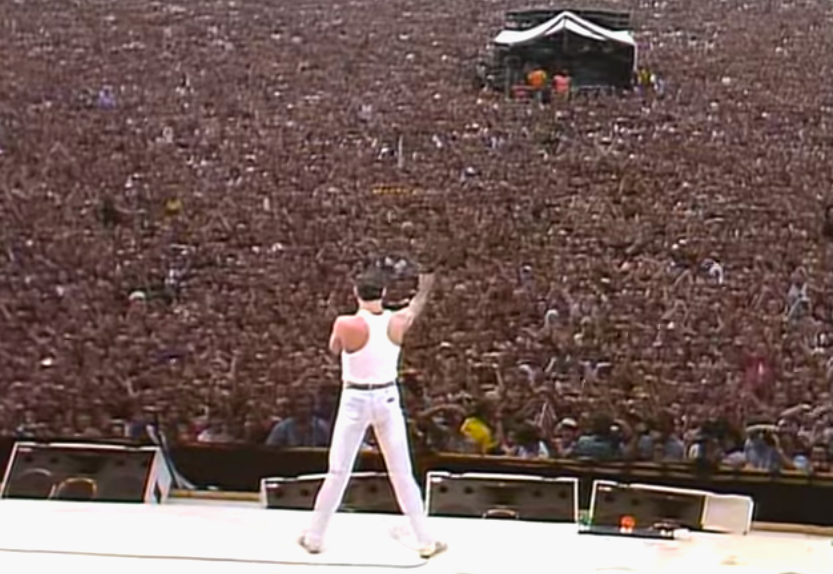This color photograph captures an electrifying moment at what appears to be Queen's set during the Live Aid Benefit concert in the 1980s, with Freddie Mercury commanding the stage. Freddie, seen from behind, dons a white tank top with a racer back and bright blue jeans, while standing with his legs spread wide apart in a V-shape. His right arm is raised triumphantly in the air, and his left hand, not visible, likely holds a microphone to his face. In front of him, numerous rectangular sound equipment and amps are positioned, directing sound towards the vast, packed crowd. The immense audience stretches out in a sea of indistinguishable faces, creating a blurry brownish mass interspersed with occasional splashes of color. A tent-like structure is set up far off in the crowd, faintly revealing two men in orange. The scene is devoid of text, animals, or other band members, focusing solely on Freddie Mercury and the euphoric energy of the moment, reminiscent of an iconic outdoor music concert like Woodstock.